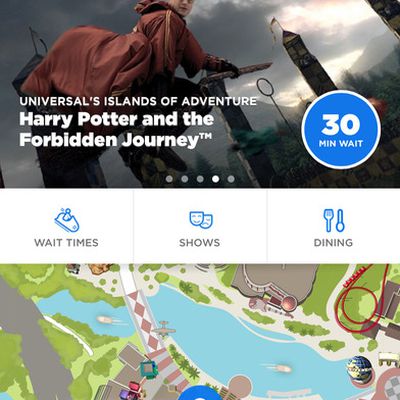Caption: 
At Universal's Islands of Adventure, near the Harry Potter and The Forbidden Journey attraction, there is a prominent display indicating a 30-minute wait time within a large blue circle. The surrounding area features a person seemingly engaged in Quidditch, wearing a red cloak and riding a broomstick. Central to the display is a wait times board, where an individual appears to be seated on something with various icons indicating nearby attractions and amenities.

The dining section is marked by a blue icon featuring a fork and spoon, signifying a nearby dining area adjacent to a river with boat rides passing under a central bridge. Beside the path leading to the rides, lush green grass can be observed. In the top right corner, red wires are visible, suggesting nearby attractions or power lines, and there is also a depiction of a beach area with abundant greenery.

A prominent universal sphere can be seen among the buildings, and an airplane is visible flying overhead, accompanied by movement marks under the boat, indicating active rides and a bustling atmosphere.